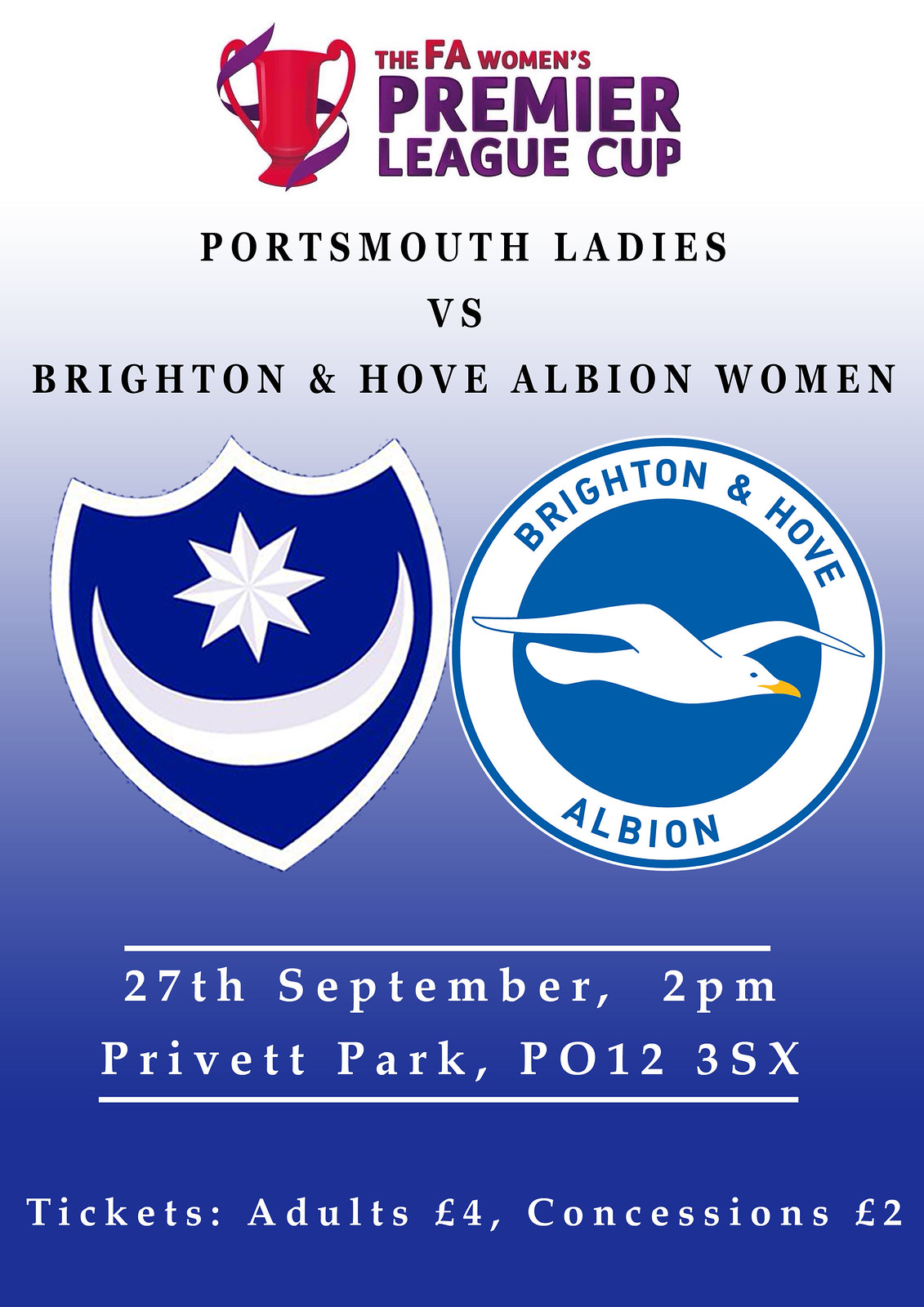This poster announces the FA Women's Premier League Cup, held on September 27th at 2 p.m. at Privet Park, P.O. 123SX. The top features a red trophy drawing with side handles, wrapped in a blue tape-like banner. To its right, red text declares "FAA Women's," followed by purple text for "Premier League Cup." Below, black text provides match details: "Portsmouth Ladies versus Brighton and Hove Albion Women," flanked by both team logos. On the left, Portsmouth's blue shield shows a white star and crescent moon. The right side features Brighton and Hove Albion's circular emblem, a blue-outlined white circle containing a flying white seagull with a yellow beak and blue eye. Ticket prices are listed at the bottom: Adults £4, Concessions £2. The gradient background transitions from dark blue at the bottom to white at the top, enhancing the layout's visual appeal.